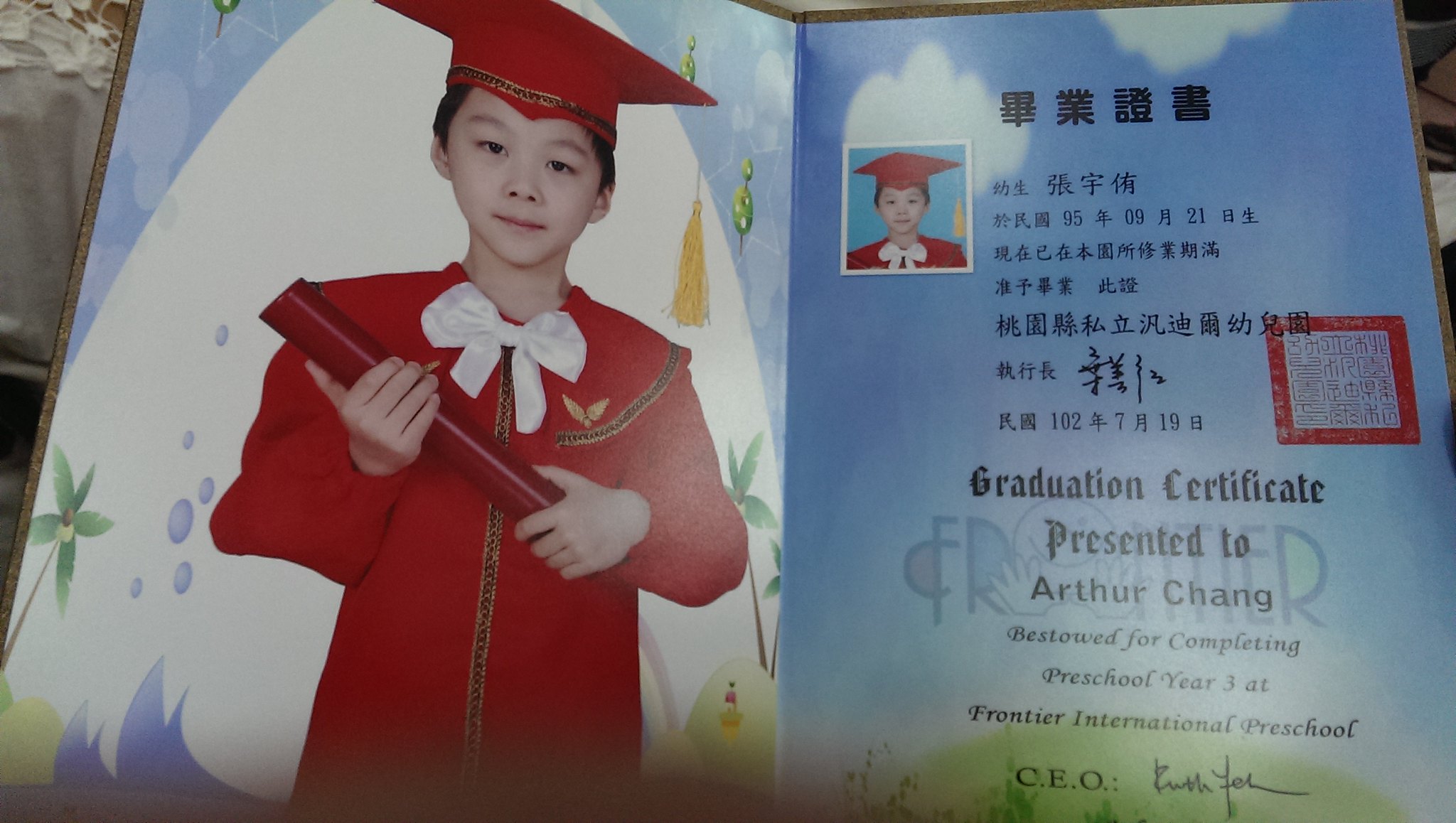This image portrays an elegant graduation card celebrating the achievement of a young boy named Arthur Chang. On the left side, a detailed photograph captures Arthur in his graduation attire. He is a young Asian boy, around six or seven years old, with brown eyes and clear skin. He is adorned in a red graduation cap, complete with a yellow tassel hanging down the right side, and a red gown complemented by a white bow tie. Cradled in his hands is a round red diploma, positioned in line with his left shoulder.

The backdrop of this photograph features whimsical elements including a white egg-like object dotted with blue spots and surrounded by green leaves, along with palm trees, purple bubbles, and flowing purple water, all set against a sky-blue background with scattered white clouds.

On the right side of the card, a small photo cutout of Arthur's face is framed by a booklet filled with bold characters from a foreign Asian language, potentially Chinese. Surrounding a red box in the center, which resembles either a QR code or additional foreign text, is a formal inscription in English: "Graduation Certificate, presented to Arthur Chang, bestowed for completing Preschool Year 3 at Frontier International Preschool, CEO Ruth Forer." The right page also features the emblem of Frontier International Preschool faintly visible in the background along with elements of green grass and white clouds.

This beautifully designed graduation card not only honors Arthur's preschool graduation but also incorporates culturally rich and visually appealing elements that add to its significance.